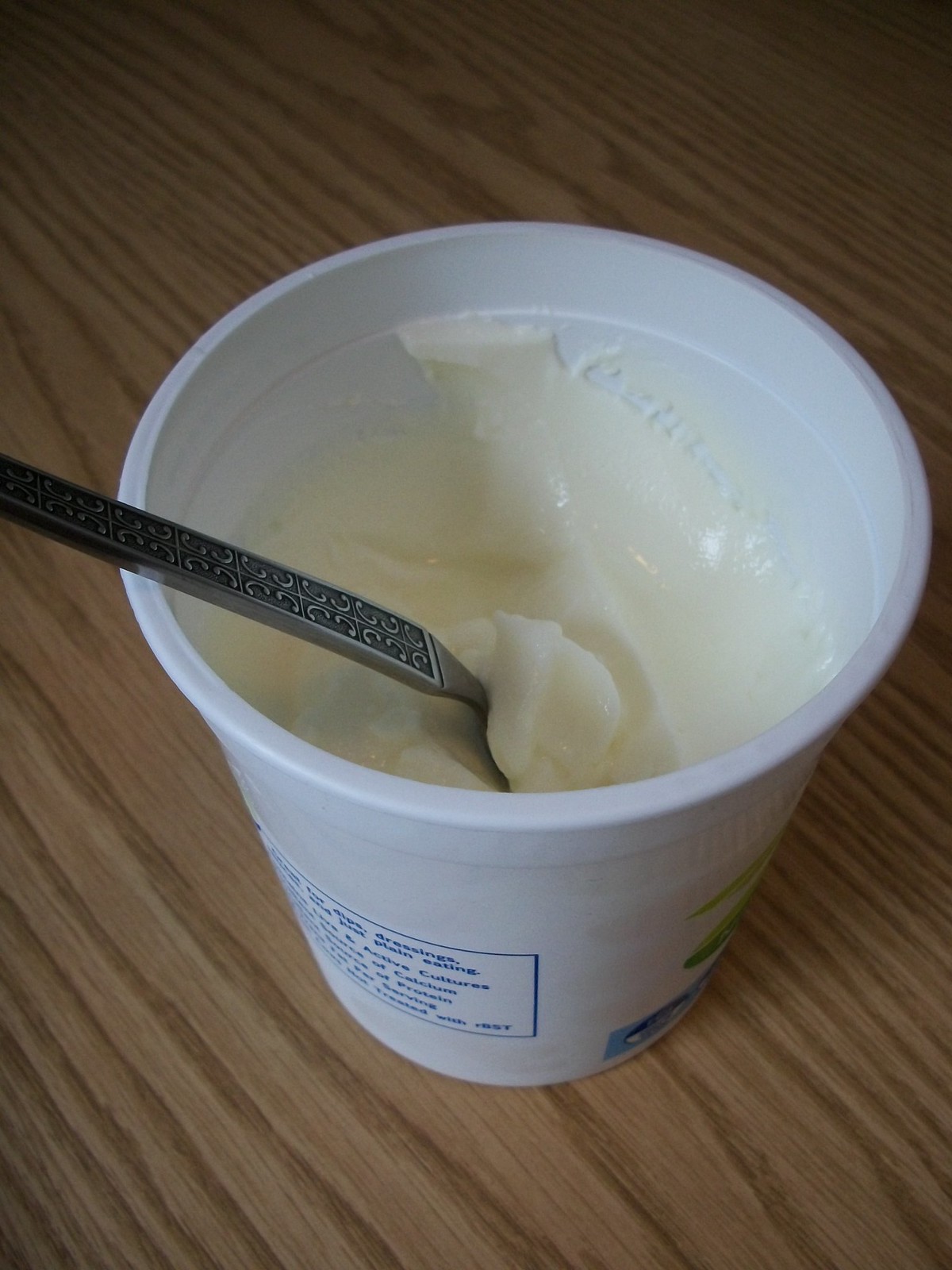This is a detailed photograph of a white plastic container, approximately four inches tall and of similar diameter, filled with a white, gelatinous substance that could be yogurt or mayonnaise. The container, positioned on a wooden countertop, features a blue rectangle with various words on the back. Inside the container, about a third of the substance has been removed, leaving two-thirds remaining. A silver spoon with an ornate handle is partially submerged in the thick, white substance, with its head buried and the body, showcasing intricate gray details, visible above the surface.